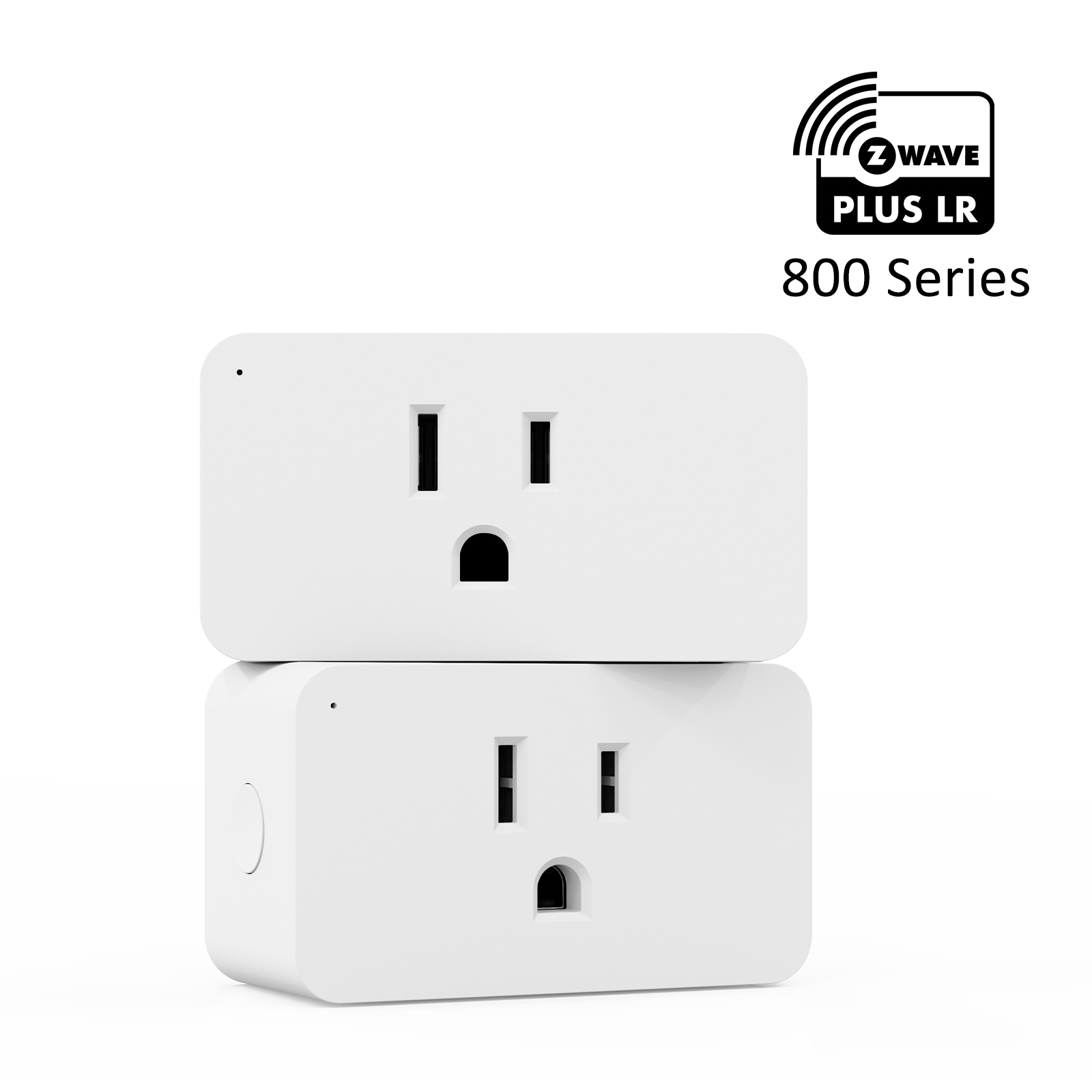The image showcases two white, portable Z-Wave Plus LR 800 Series electrical sockets, stacked one on top of the other. Each socket features a three-pronged outlet reminiscent of faces, with the top outlet appearing as if it has two eyes and a mouth, and the bottom outlet leaning slightly to the right. On the left side of each outlet, there is a small circular button. At the top of the image, a logo is displayed within a rectangular outline; the upper half of the rectangle is white with black text reading "Z-Wave" and accented by a sound wave symbol emanating from the "Z". The lower half of the logo is black with white text that says "PLUS LR" followed by "800 SERIES" in black text beneath it.